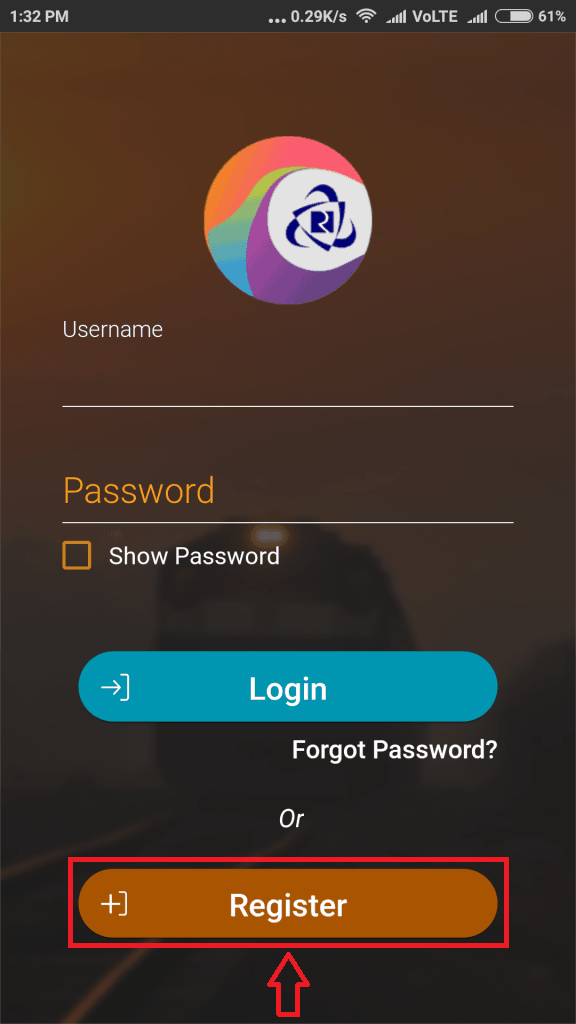This is a detailed screenshot taken from a smartphone, portraying a login page with a dark, chocolate brown background. The screen features interactive elements, including a prominent blue button for logging in, which has "Login" inscribed in white font. Beneath it, there's an option that reads "Forgot password," followed by the word "or." Adjacent to this, a burnt orange rectangle serves as the registration button, labeled "Register." This button is accentuated by a red triangle pointing towards it, accompanied by an upward arrow icon.

The page contains input fields for the user’s credentials, with designated spaces to enter a username and password. An additional checkbox allows users to choose whether to display the entered password.

At the top of the page, a distinctive logo captures attention. It consists of a swirling circle with blended hues of red, blue, purple, and green. The center of this swirl features a smaller white circle embedded with a black design. Although faint, a background image provides a subtle depth to the overall layout.